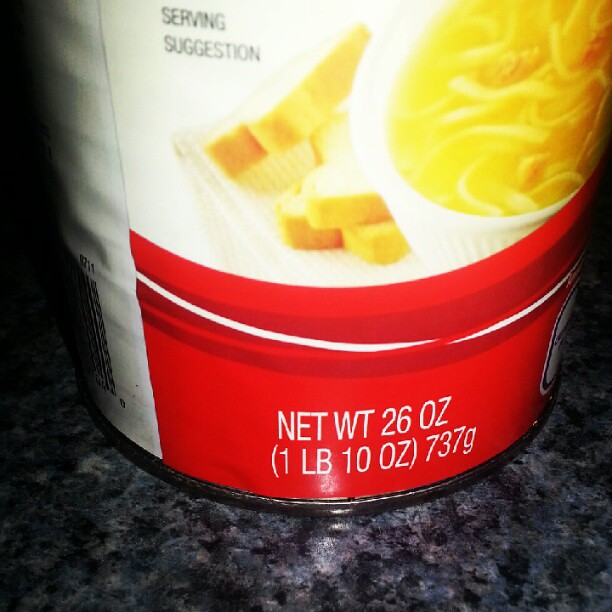The image features a container of soup, prominently displaying the text "Serving Suggestion" near the top. At the bottom, it states, "Net Weight: 26 oz (1 lb 10 oz) 737 g." The container appears to be designed for chicken noodle soup, with an appetizing image of the soup and some bread behind it on the label. The container itself has a white top and a red bottom label. It is placed on a dark-colored kitchen counter that appears to be a mix of black and silver tones. On the upper right side of the container, a small portion of the barcode is visible. Overall, the setting suggests a pre-preparation stage in a kitchen environment, with the soup container being the primary focus of the image.